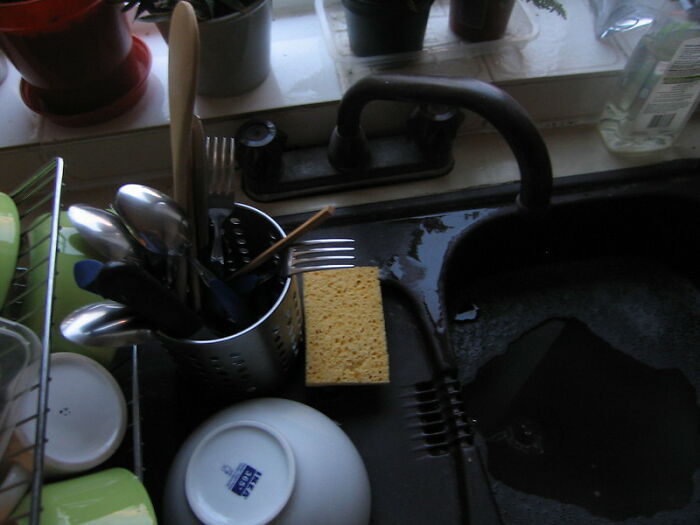This image features a sleek, black sink paired with a matching black tap. Behind the tap are coordinating black handles set against a backdrop of a white tiled ledge. This ledge is adorned with greenery, specifically two green plants resting on a plastic container. A larger plant with green foliage is positioned next to a red-hued plant on the left side of the ledge. 

On the countertop near the sink, there is an orange sponge placed beside a gray metal utensil holder. The holder is filled with silver forks and spoons and also contains a brown wooden spoon. In front of the utensil holder sits a porcelain bowl, distinguished by a striking blue square at its base. To the left of this bowl, there are two green bowls flanking a white tea or coffee mug. Leaning against these items is a metal dish rack that supports another green bowl and a plastic lid. To the right side of the sink, a clear plastic bottle with black font detailing its contents is filled with a transparent liquid, adding a functional touch to the scene.